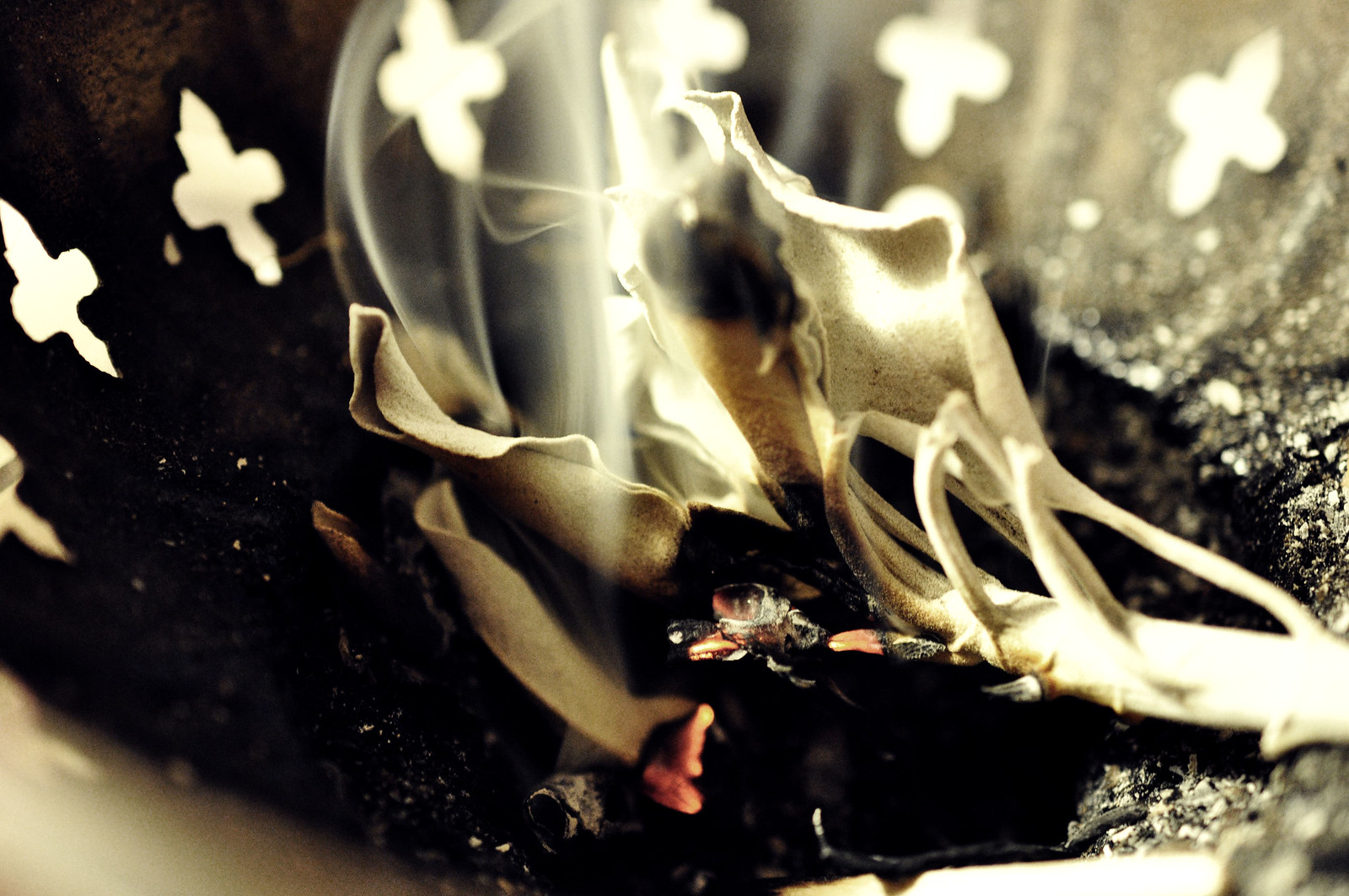This photograph is a close-up image of a metallic, black bowl with small, cross-shaped cutouts around its sides. Inside the bowl, a white paper is burning, emitting wisps of smoke as not all of it has fully caught fire. The paper shows varying stages of combustion: some parts have turned black, others have become brown, while a substantial portion remains white. Red embers are visible at the edges of the burning paper. Beneath the lit sections, charred remnants and ash are evident. The image captures the transitory beauty of the burning paper in a rectangular frame.